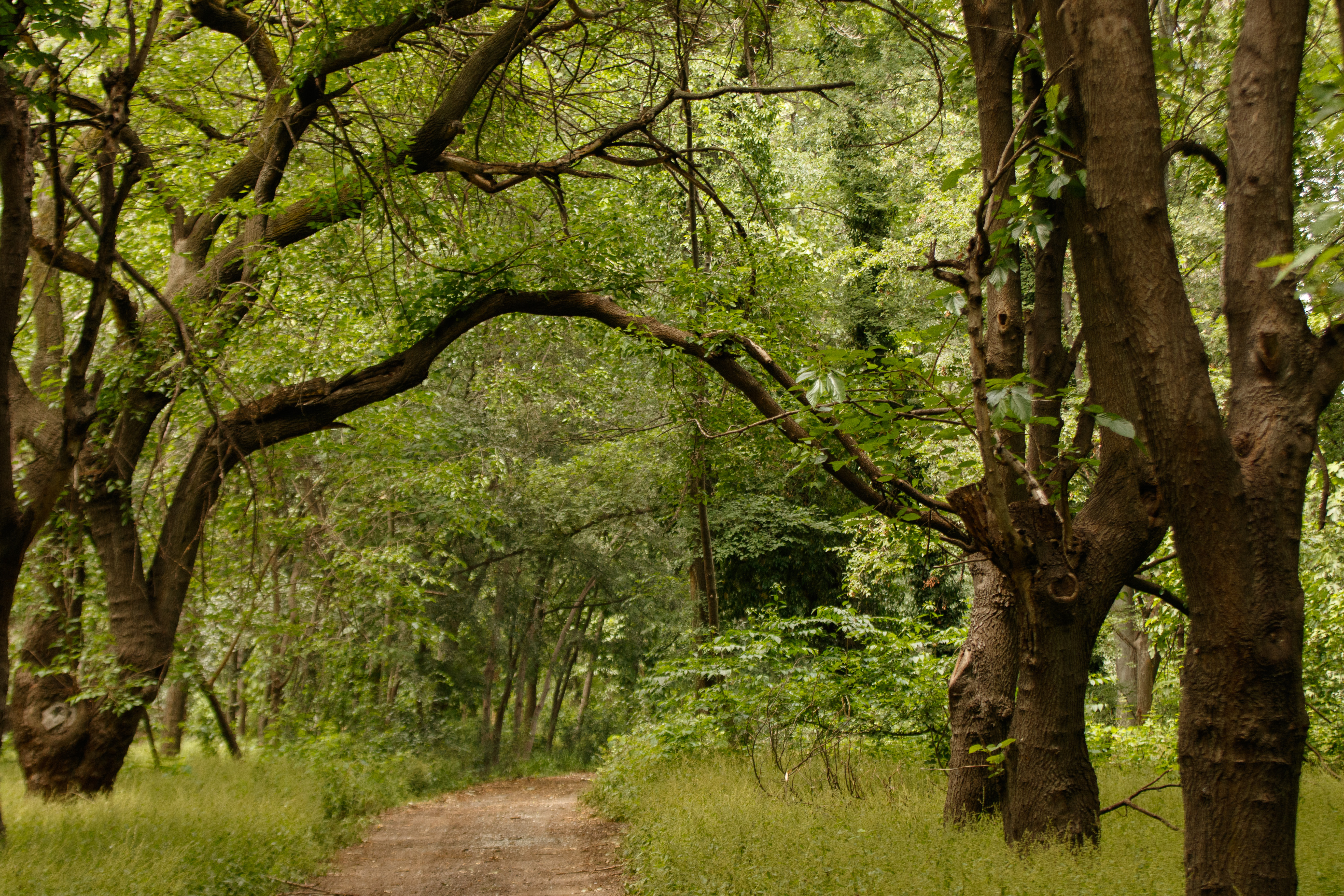The image depicts a forested trail winding through a verdant, wooded area. Dominated by a mix of large and medium-sized trees, the scene showcases two towering trees to the right and a particularly striking tree to the left with thick, long branches spreading out in all directions and adorned with lush green leaves. The forest canopy forms a sort of tunnel over a brownish-tan earthen path that stretches from the bottom left corner of the image and disappears into the dense growth of smaller trees in the distance. Sunlight gently filters through the leaves, casting dappled shadows on the ground. The path itself is a mix of gravel, stone, and dirt, flanked by high grass and shrubs. Here and there, little knobs and growths can be seen on the trees, where limbs have started to grow and fallen off. The scene is devoid of people or animals, exuding a tranquil, secluded atmosphere ideal for hiking and exploring nature.